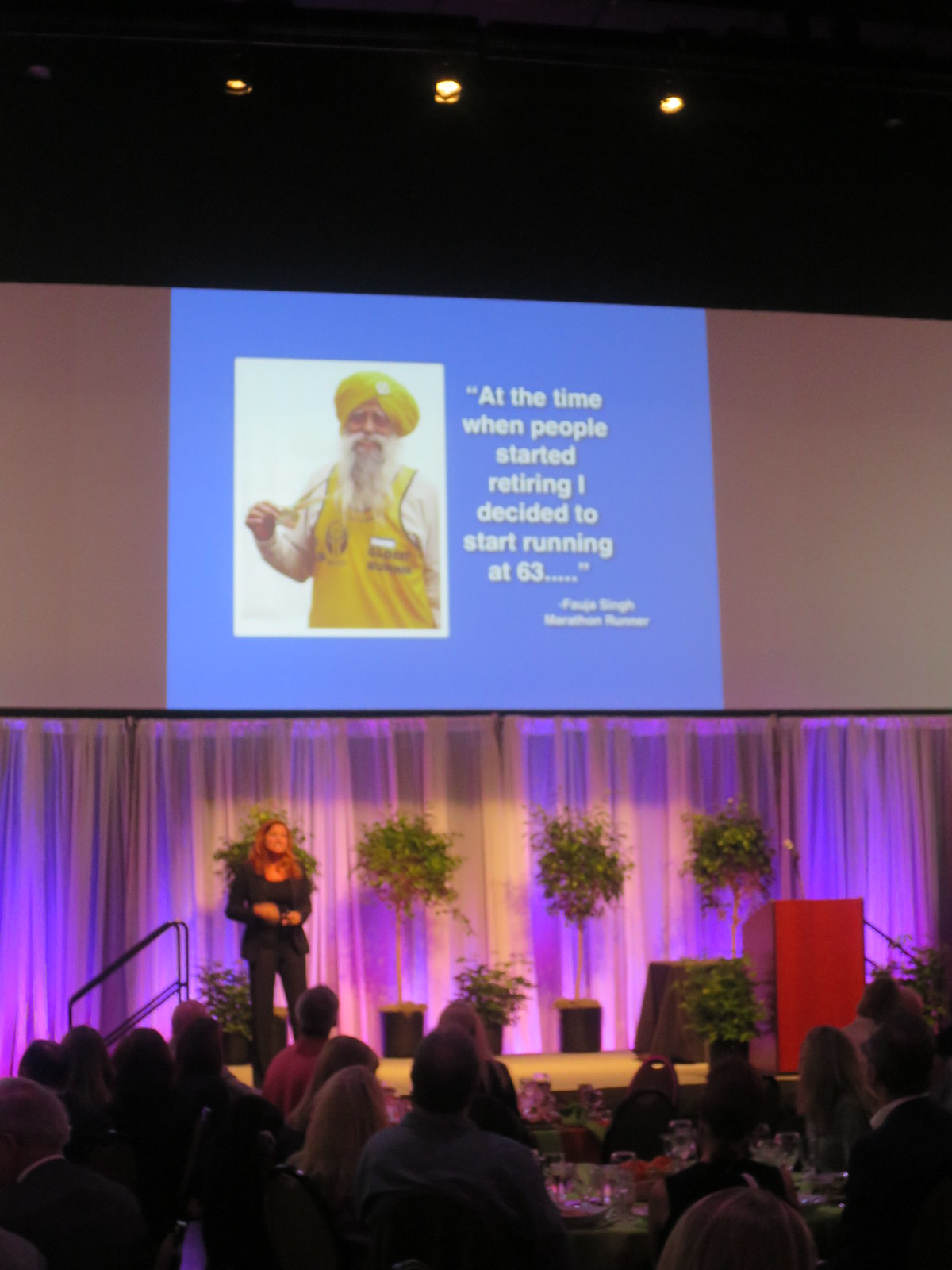The image depicts a speaking event set in a catering hall, illuminated by purple lights with white drapery as the backdrop. Centered on the stage is a woman with long brown hair, wearing a long black sleeve shirt and black pants, delivering a speech to an audience seated at banquet tables adorned with glasses and plates. She stands beside a wooden podium equipped with a microphone but isn't using it as she moves around the stage, which also has stairs and several potted fake trees. Above her is a projector screen displaying a South Asian man in a yellow turban and yellow attire, accompanied by the quote, "At the time when people started retiring, I decided to start running at 63." The top portion of the image features a black bar and three lights in the upper left, center, and right, illuminating the scene below. The foreground captures the back of the audience's heads, attentively watching the speaker.